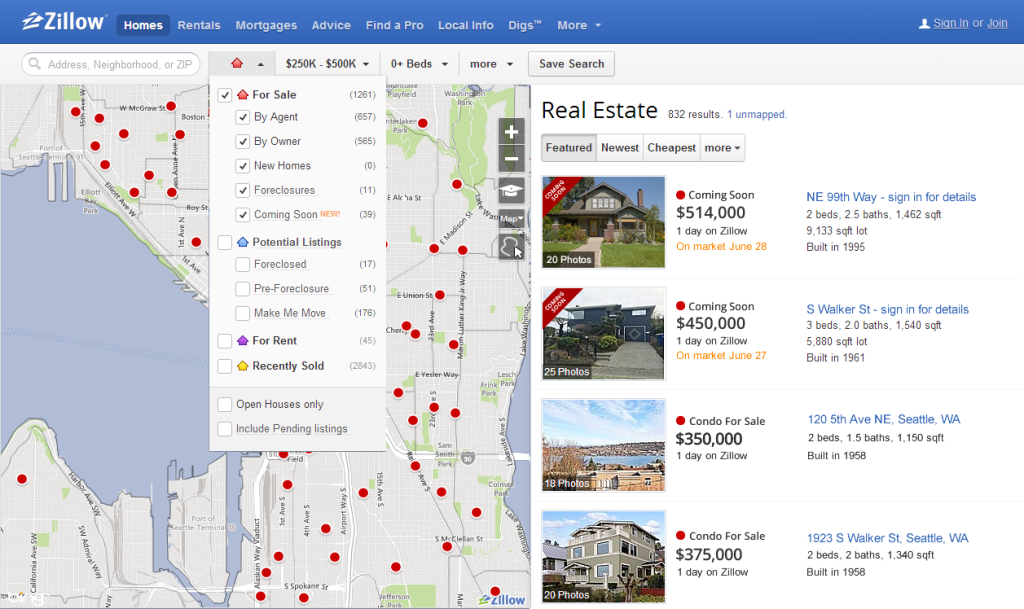The screenshot captures a Zillow website interface, prominently displaying the Zillow logo in the upper left corner. Adjacent to the logo, the navigation menu lists various categories: Homes, Rentals, Mortgages, Advice, Find a Pro, Local Info, Digs, More, and options to Sign In or Join. 

Below the navigation bar, a detailed map with numerous red dots marking property locations is visible. The map overlays a search filter dropdown menu offering options such as For Sale By Agent, By Owner, New Homes, Foreclosures, Coming Soon, Potential Listings, Foreclosed, Pre-Foreclosure, Make Me Move, For Rent, Recently Sold, Open Houses Only, and Include Pending Listings.

To the right of the map, a property listing section highlights individual homes. The first listing displayed is a property priced at $414,000 with a note indicating it was listed one day ago on Zillow, having entered the market on June 28th. The overall screenshot provides a comprehensive view of the Zillow website's real estate search functionalities and current listings.